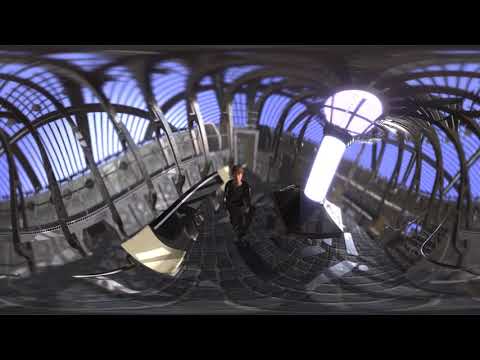The image is a horizontally oriented, slightly blurry, rectangular picture with a distinct, thick black border at the top and bottom. The central scene appears to be computer-generated and evokes a fantastical, almost sci-fi ambiance reminiscent of a Star Wars spacecraft interior. The lower part of the structure consists of gray walls with gray arched support beams extending upwards. The upper sections feature vertical strips of blue, through which light filters into the room. There is a central column crowned with a bright, white glowing dome or orb that resembles a giant light bulb, likely serving as the focal point of illumination.

An indistinct character, possibly a person, appears in the center of the image, dressed in black with short brown hair, though their details are obscured due to the blur and potential fisheye lens distortion. The ground is characterized by dark gray lines with thin gray outlines, giving a metallic, wavy appearance. The overall atmosphere is both mysterious and semi-realistic, enhanced by the light playing off various elements within the space, including the metal plates that form the floor.